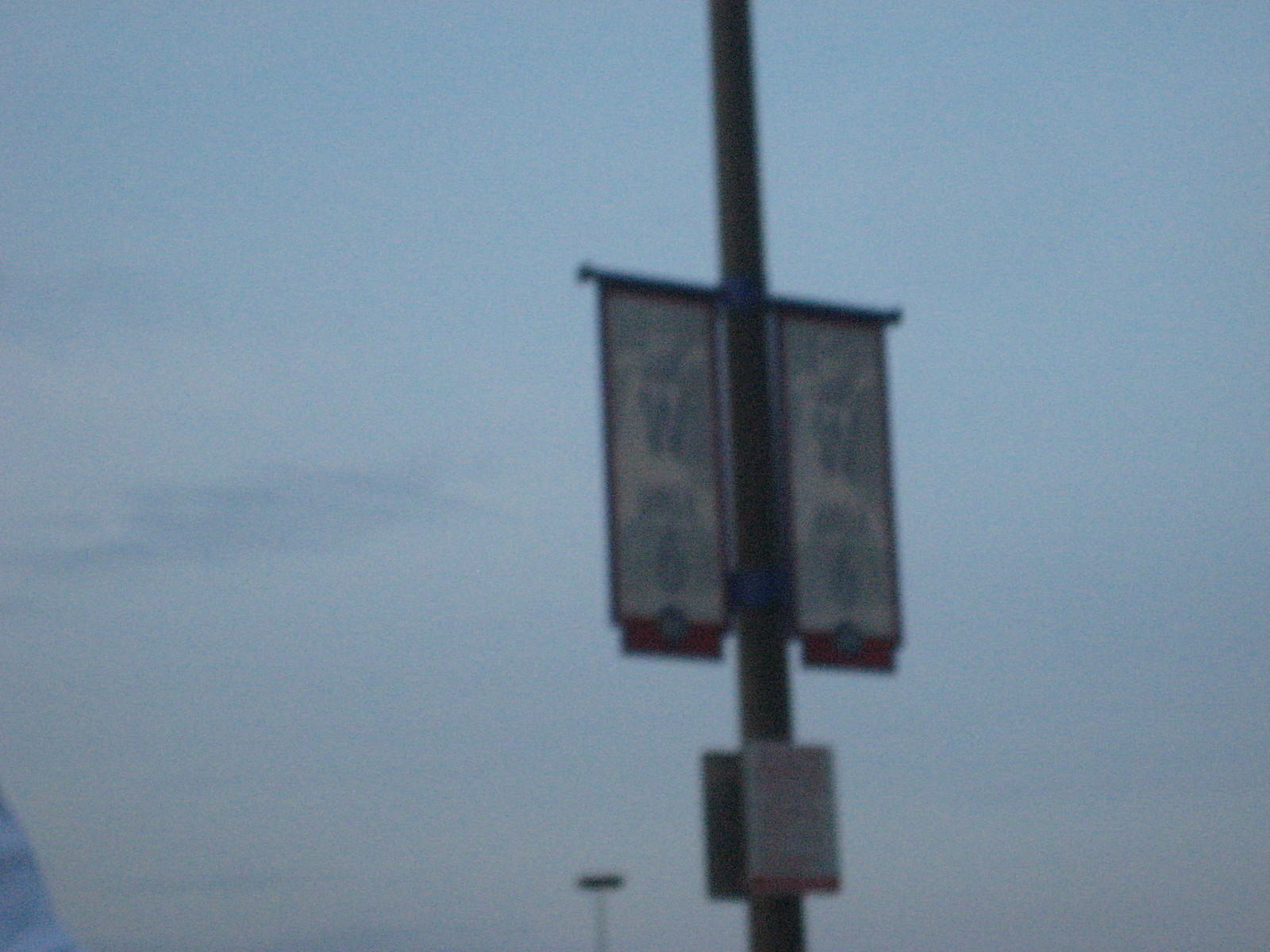This is a blurry photograph taken at nightfall. In the foreground, there is a pole with two twin banners attached to it. Both banners are white with blue writing, displaying the letter 'W' followed by the number '6' beneath it. Further down the pole, another white sign with a red banner across the bottom is visible, although the text is unreadable. The background reveals a mostly clear sky with a few stray clouds scattered in the distance. Additionally, another small, indistinct sign is mounted high on a distant pole, too far away to be legible.